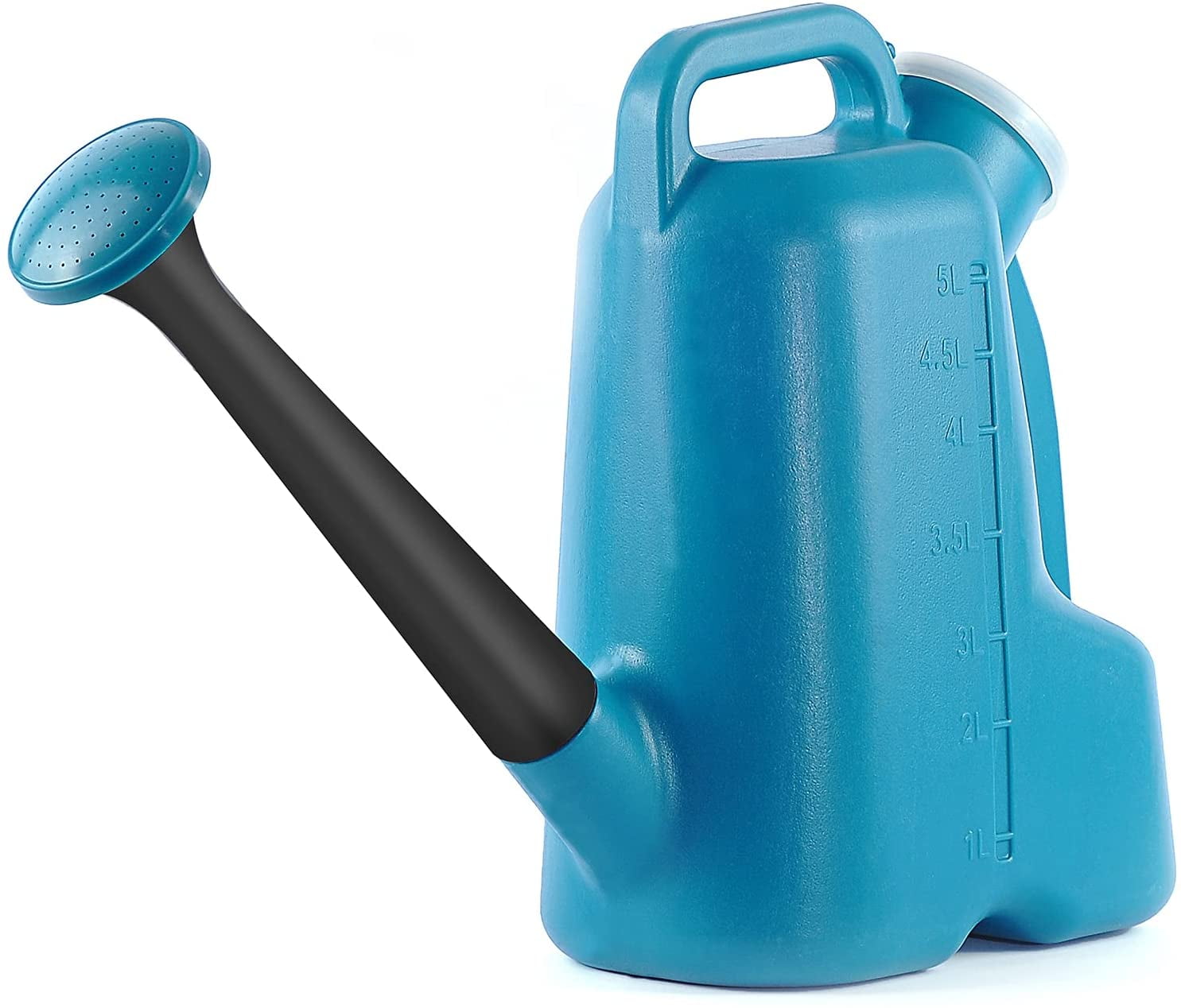This image depicts a large, predominantly blue plastic watering can. The can is more tall than it is round and features a long, black spout extending from the bottom left side, culminating in a blue circular sprinkler with tiny holes for water dispersion. The top of the can is equipped with a sturdy blue handle. Positioned to the right of the handle is a translucent lid for water filling. One side of the can bears a vertical measurement scale, marked in liters, displaying increments from 1L through 5L, including half-liter measurements at 3.5L and 4.5L. The design is both functional and straightforward, with no additional text or imagery.